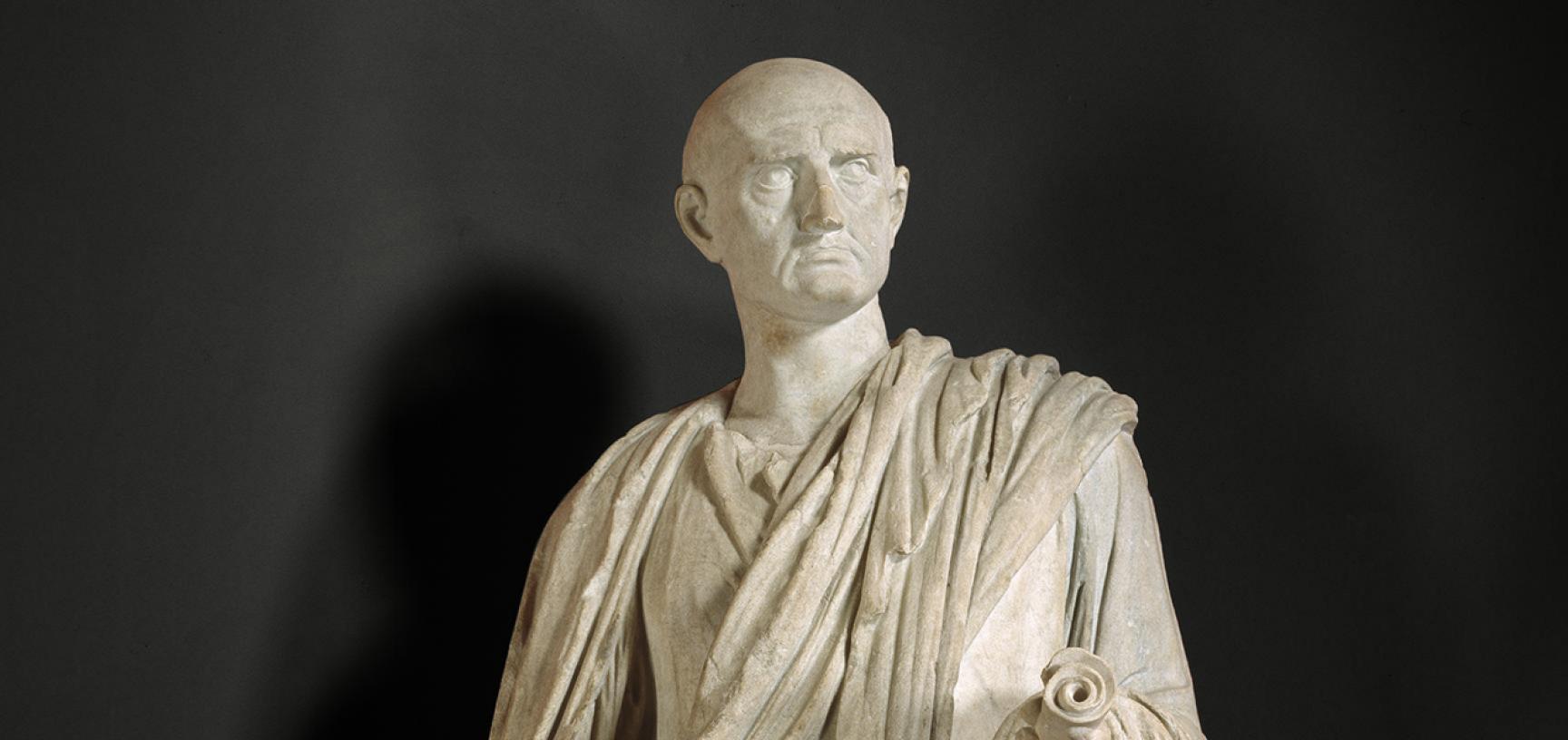This detailed image captures an ancient-looking marble statue set against a stark black background, emphasizing the intricate craftsmanship. The statue depicts a bald man, facing slightly off to the side with a stern, almost concerned expression. His brows are furrowed, revealing subtle forehead wrinkles, while additional lines frame his mouth, and a notable mole rests just below his right eye (to the left in the image). His attire features a draped fabric, resembling a toga or sash, over his left shoulder, adding to the classical feel of the sculpture. Held in his left hand is what appears to be a rolled-up scroll or document, suggesting a figure of importance, perhaps from ancient Greek or Roman times. The statue’s faded white and tan hues enhance its aged appearance, completing this finely detailed historical portrayal.